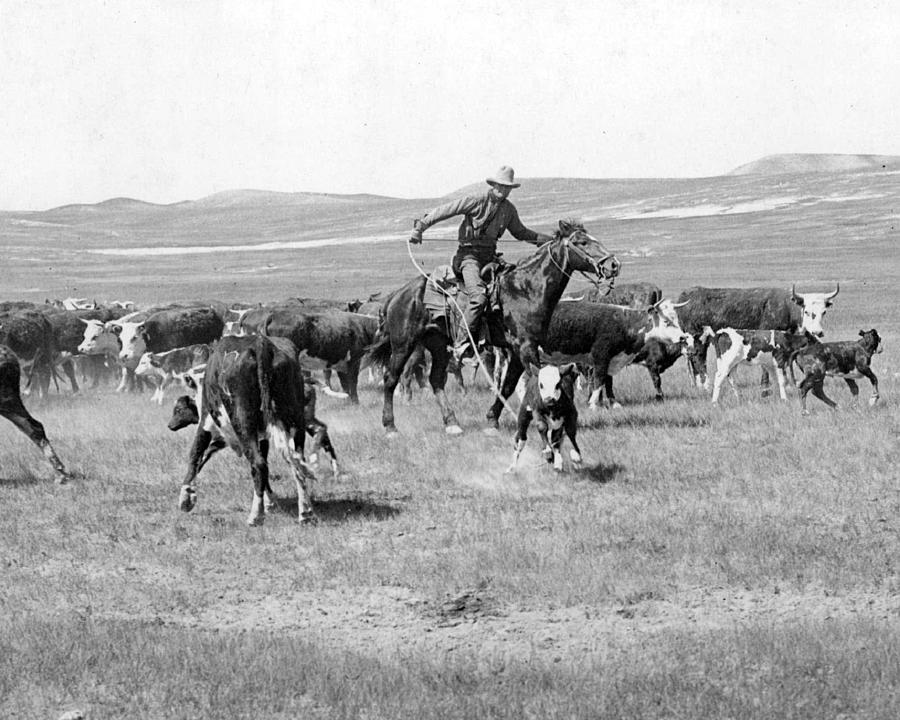A timeless black and white photograph captures the essence of a bygone era, portraying a desolate farming landscape with gentle, rolling hills lining the horizon. Centered in the frame, a rugged cowboy sits astride a sturdy horse, exuding a sense of calm amidst the chaos. Donning a traditional cowboy hat, he firmly grips a coiled rope, embodying the iconic figure of a cattle herder. Surrounding him, numerous cows of diverse shapes and sizes scatter in all directions, their movements frenetic and seemingly panicked. The stark contrast of the monochrome palette accentuates the raw intensity and dynamism of the scene, evoking a powerful impression of life on the range.